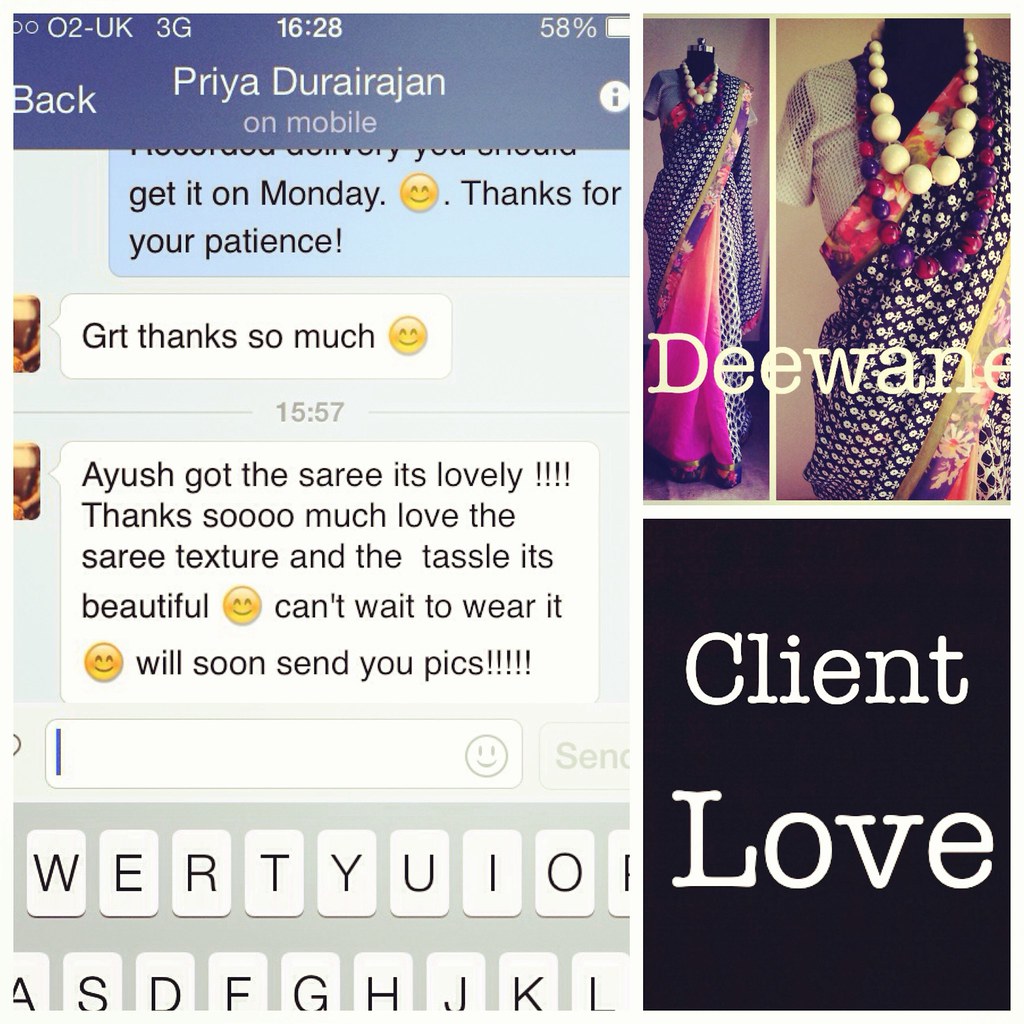This image is a collage showcasing client appreciation and features two primary sections. On the left, there's a detailed screenshot of a Facebook Messenger chat between Priya Durai Rajan and another person. The conversation expresses gratitude and admiration for a sari, with messages like "Thanks for your patience" and “Ayush got the sari, it’s lovely, love the sari texture and the tassel, it’s beautiful, can't wait to wear it.” Above the chat, the phone displays details such as the network "0-2 UK 3G" with a time stamp of "16:28" and a battery level at "58%."

On the right side of the collage, there is an image of a traditional sari displayed on a mannequin, accessorized with a designer necklace. The top right corner of this side features the watermark “Diwane,” likely indicating the brand. Below this image, a black background bears the words "client love" in white text, emphasizing the appreciation aspect of the collage. The overall colors observed in the image include dark blue, white, light blue, yellow, gray, pink, red, and tan, contributing to a vibrant and engaging visual presentation.